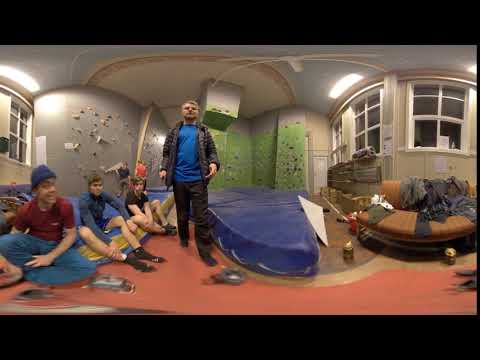The image depicts an indoor room featuring a mix of green and gray walls, with the green wall at the back and the gray ones on the sides. The right side of the room showcases several windows. The flooring is covered with an orange-colored rug, and various mats are present on the floor, including a cushiony blue one. On the left half of the picture, there are four individuals: three young boys sitting on the floor and a man standing beside them. This man, positioned near a couch or foam seating structure, is wearing a blue shirt layered under a black jacket and paired with black pants, appearing to be barefoot. The image suggests an informal, relaxed gathering, possibly involving friends engaging in activities such as playing video games. Notably, the photo exhibits signs of warping, implying that a VR or 360-degree lens was used, leading to some distortion, particularly visible in the stretched appearance of the couch-like bench on the right side.